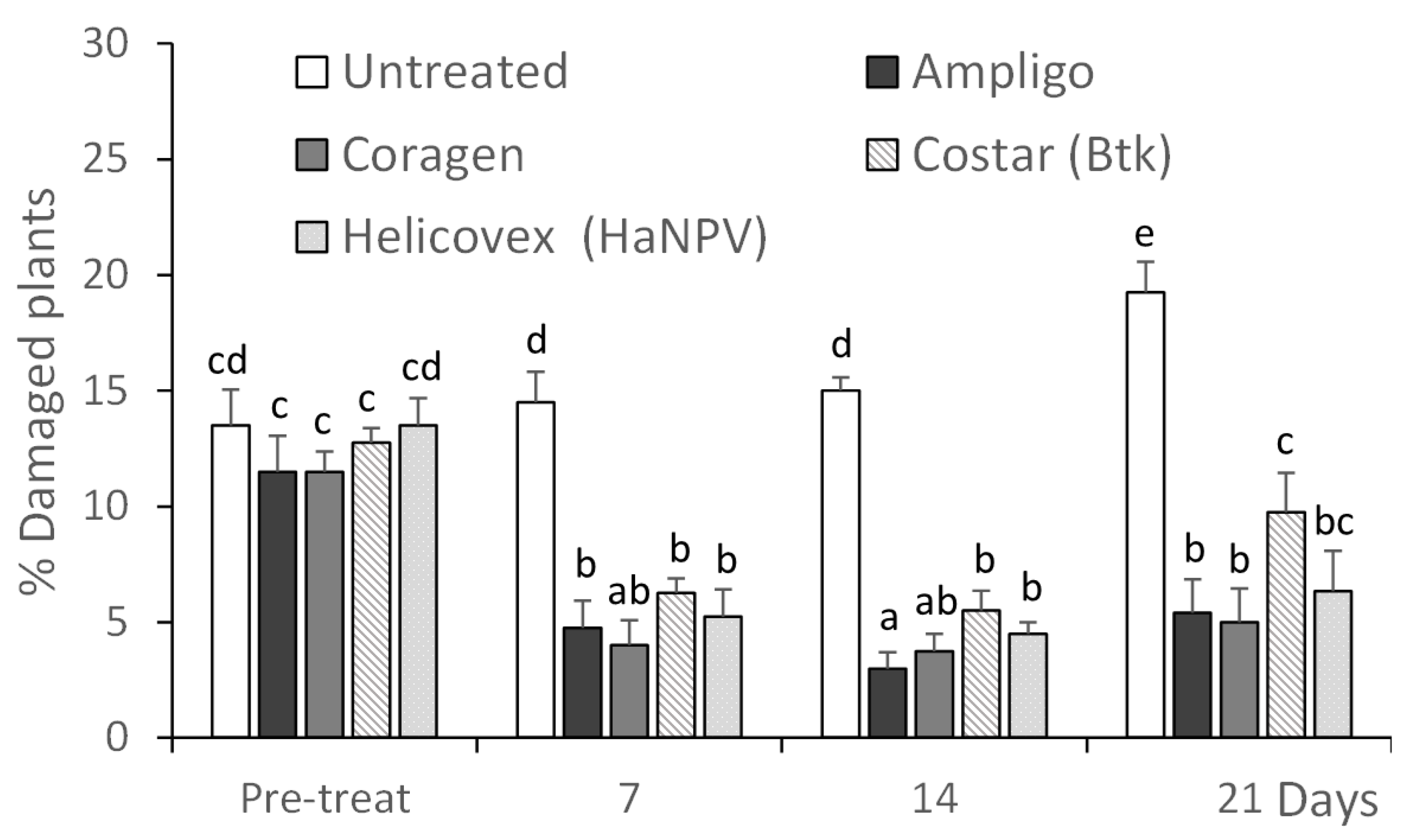The image is a square, black-and-white bar graph with a white background. Along the left side, there is a vertical y-axis labeled "Percentage of Damaged Plants," with a scale ranging from 0 to 30. The bottom x-axis shows four time points: "Pre-treat," "7 days," "14 days," and "21 days." 

Each time point includes several bars representing different treatment options: untreated, corrigin, halicovics, ampligio, and costar. The treatments are distinguished by varying shades and patterns: clear for untreated, dark for corrigin, gray for halicovics, black for ampligio, and gray with stripes for costar. 

The bars' heights indicate the percentage of damaged plants at each time point, visually illustrating the effectiveness of each treatment over time. The image likely comes from a study, report, or textbook on horticulture, showing how different insecticides affect plant damage over a 21-day period. Each treatment's performance is immediately apparent, with untreated plants generally showing higher damage percentages compared to treated ones.